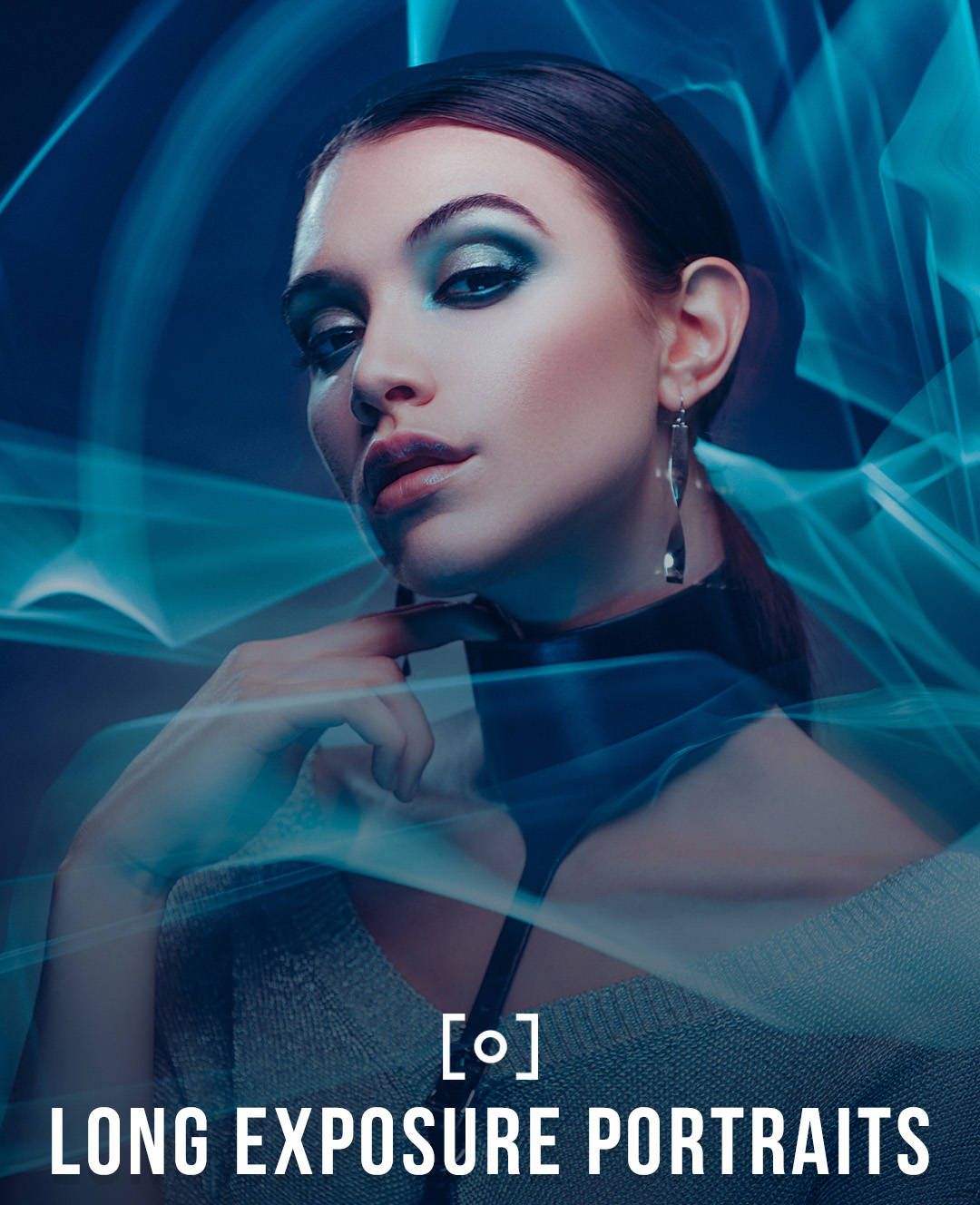This highly striking and professionally posed photograph features a brunette model with her hair styled into a sleek ponytail, set against a dark blue background. She exudes a futuristic aura, with heavy blue eyeshadow that enhances her sharp, arched eyebrows, along with perfectly applied brows and lipstick. Her icy, cyber-themed makeup and the swirling, gauzy light effects around her suggest a specialized "long exposure portraits" technique, emphasized by the white text at the bottom of the image. 

The model is adorned with long, glittering silver earrings and a woven gray sweater beneath a black leather collar, which has an attached strip running down her chest. Her right hand delicately touches the collar, as she gazes alluringly at the viewer with her head slightly tilted to the right, lips parted. The entire photo carries a blue and teal tint, amplifying its futuristic and editorial vibe. There is a symbol above the text, consisting of two bracket signs enclosing a circle, potentially indicating a logo. This evocative image could likely be part of a fashion editorial, a modeling portfolio, or a tutorial showcasing advanced photography techniques.